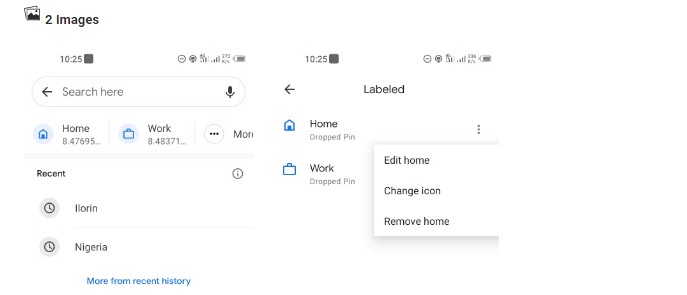In this image, we can see a close-up of a computer interface focusing on a search bar and related functionalities. At the top left corner, there is a section labeled "Two Images," which is followed by the number "1025." Adjacent to these, a few icons are visible, including one that resembles airplane mode, a power symbol, and Wi-Fi strength indicators. The number "1025" appears again beside a black square similar to the one under "Two Images."

On the left-hand side, below these symbols, there is a search bar labeled "Search here" accompanied by a microphone icon. Below the search bar, there are location tags: "Home" with the coordinate number "8.47695," and "Work" with the coordinate number "8.48371." Next to the work coordinate, there is an assumed date labeled "Monday," followed by a small circular symbol containing three dots.

Further down, there is a "Recent" section displaying the words "Leorin" and "Nigeria." Next to this is a labeled section containing "Home dropped pin" and "Work dropped pin." The options "Edit Home," "Change Icon," and "Remove Home" are also visible within a white box.

This detailed depiction captures the intricate layout and functionality of the computer's search interface.